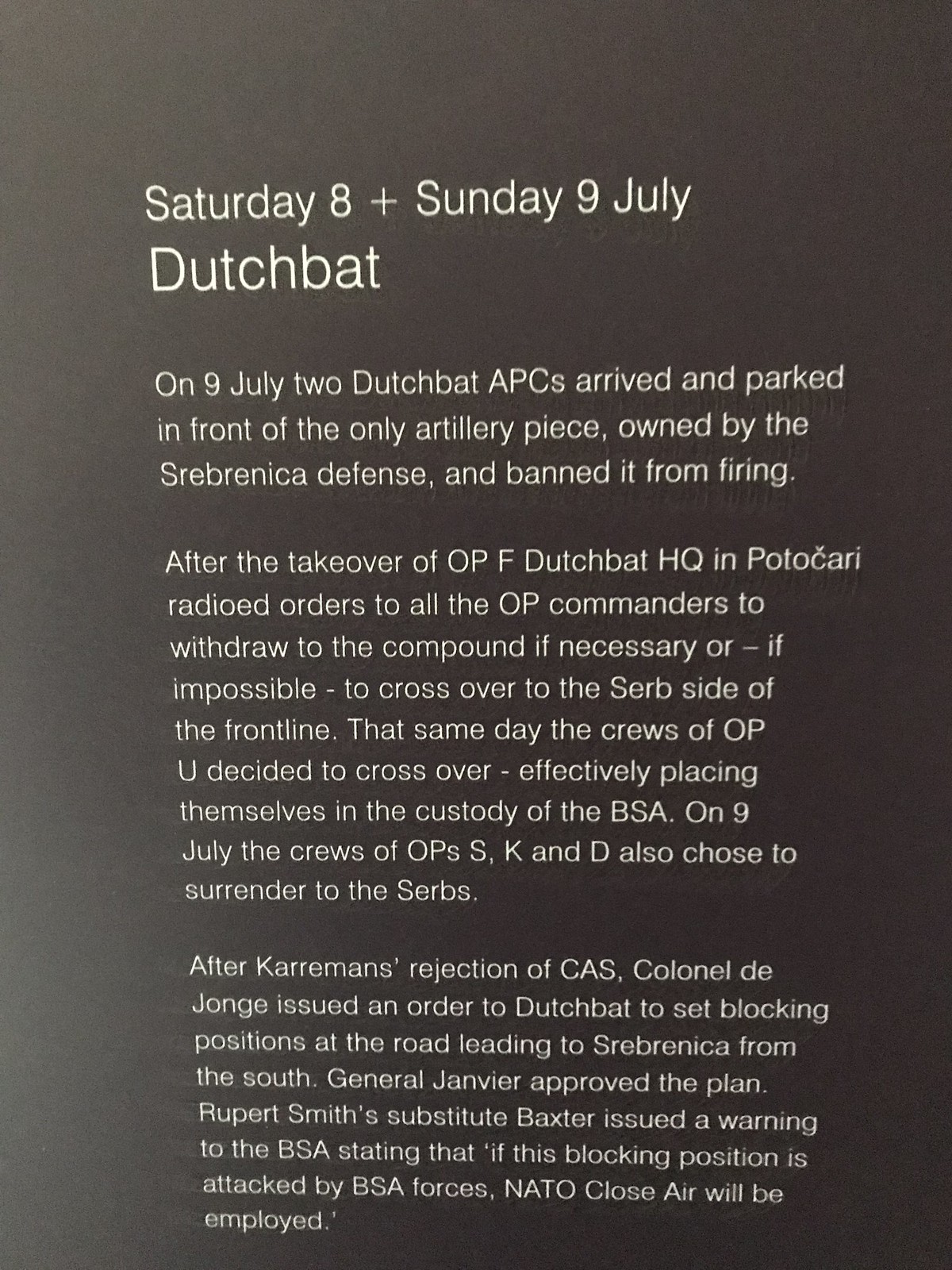In a white-on-deep-gray backdrop, the text at the top of the image reads: "Saturday 8th plus Sunday 9th July Dutchback." Below, it provides a detailed account: On July 9th, two Dutchback APCs arrived and strategically parked in front of Srebrenica's sole artillery piece, effectively banning its use. In the wake of OPF's takeover, the Dutchback HQ in Potocari issued urgent orders via radio for all OP commanders to withdraw to the compound or, if necessary, to cross over to the Serbian side. That same day, the OPU crews decided to cross over, thereby surrendering to the BSA's custody. Additionally, the crews of OPSSKND also chose to yield to the Serbs. Following Karaman's rejection of close air support (CAS), Colonel De Jong instructed Dutchback to establish blocking positions on the road leading to Srebrenica from the south, a plan endorsed by General De Jong. Baxter, Rupert Smith's substitute, cautioned the BSA that any attack on these blocking positions by BSA forces would prompt a NATO close air support response.